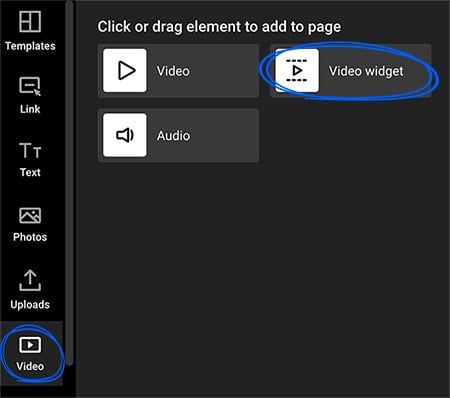A screenshot of a minimalistic user interface is displayed against a simple black background. The left side features a vertical navigation panel with icons and text labels for "Templates," "Link," "Text," "Photos," "Uploads," and "Video." The "Video" option, represented by an equilateral triangle icon pointing to the right, is circled to indicate selection. 

On the right side of the screen, there is a message prompting users to "Click or Drag Element to Add to Page," offering options such as "Video," "Audio," or "Video Widget." The "Video Widget" option is circled using a blue pencil marker, suggesting a user action. The "Audio" option is illustrated with a speaker icon emitting sound waves. 

This interface appears to guide users in customizing a website by adding or modifying multimedia elements. The overall design is clear and minimalistic, with each section represented by simple yet intuitive icons.